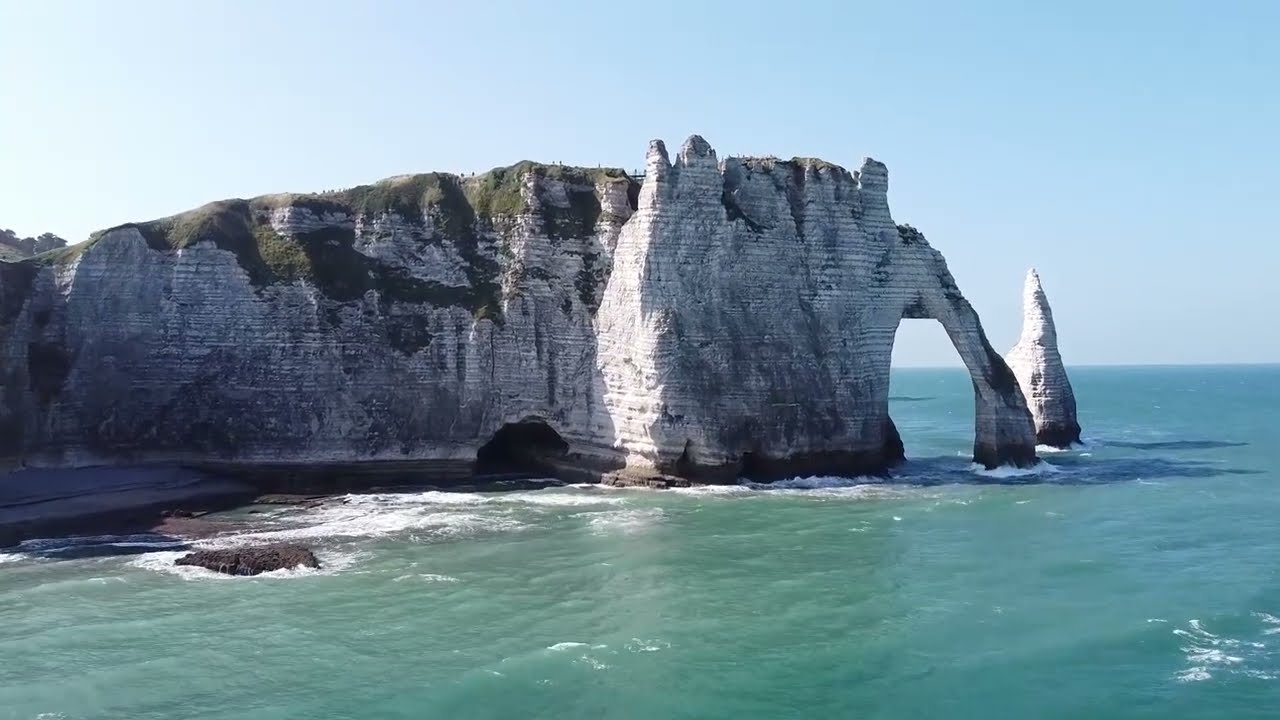The photograph captures a stunning coastal scene with a clear, vivid blue sky towering above the ocean. Central to this image is a prominent, tall white rock formation with hints of gray and black, indicative of various geological layers. The top of the rock is crowned with rich green moss, grass, and small bushes, adding a touch of verdant life to the stark structure. Wind can be sensed from the visible waves and the way the water breaks against the rock, creating foamy white splashes.

To the right side of the rock formation is a dark, intriguing cave entrance, a larger tunnel carved naturally by the elements. Adjacent to it, a smaller tunnel appears, mimicking the shape of an elephant’s trunk as it juts into the water. The turquoise and emerald hues of the water are crystal clear, reflecting the warmth of what appears to be a sunny day. On the left side of the image, a small beach cradles the scene, nestled beside the cliff walls that display distinct horizontal lines and a rough, layered texture. These natural features combine to create a tranquil yet awe-inspiring coastal landscape.